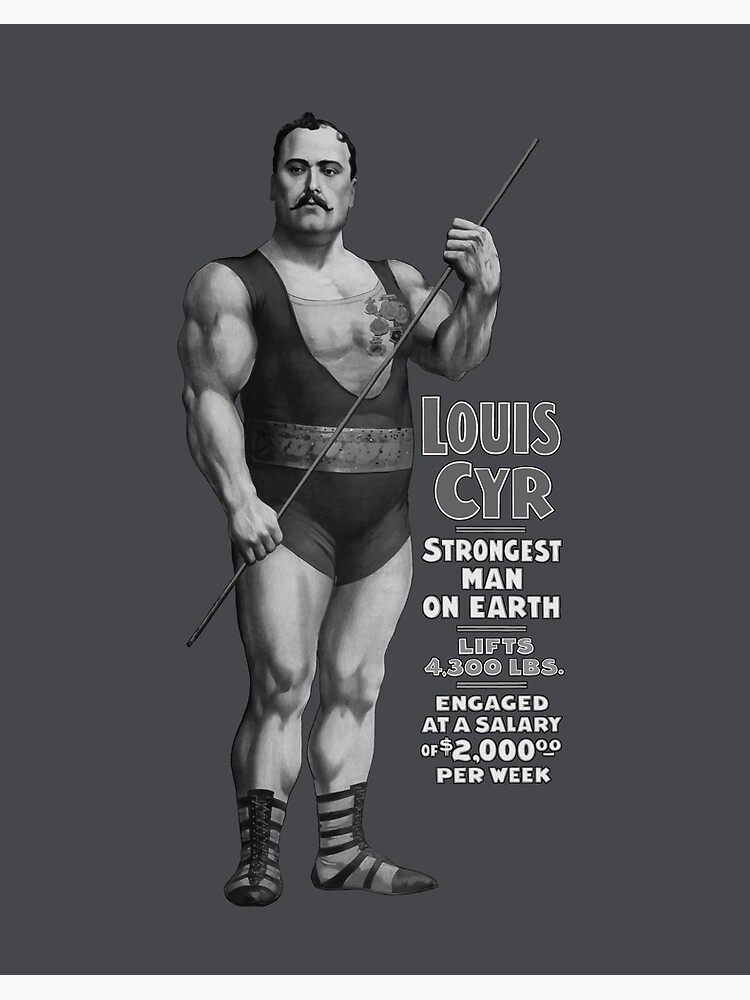This black-and-white illustration from the early 20th century depicts Louis Cyr, celebrated as the strongest man on earth. He is an imposing figure with a muscular build, a dark long mustache, and very short, dark curly hair. Cyr stands facing the camera, his body slightly angled to the right while gazing slightly left. He's clad in a dark, skin-tight unitard that covers his shoulders, paired with a colorful belt at his waist. His feet are adorned with striped, black-and-gray boxing shoes that lace up in the front. Cyr's attire is complemented by various medals displayed on his left breast.

In his hands, he holds an iron rod, which extends across his body, with his right arm stretching to the right and his left arm flexed at a 90-degree angle. The iron rod appears as though he is about to bend it, showcasing his immense strength. To the right of the strongman, bold text in gray and white states: "Louis Cyr, strongest man on earth, lifts 4,300 pounds, engaged at a salary of $2,000 per week." The monochromatic background, detailed attire, and vintage style encapsulate the early 1900s era of strongman performances.